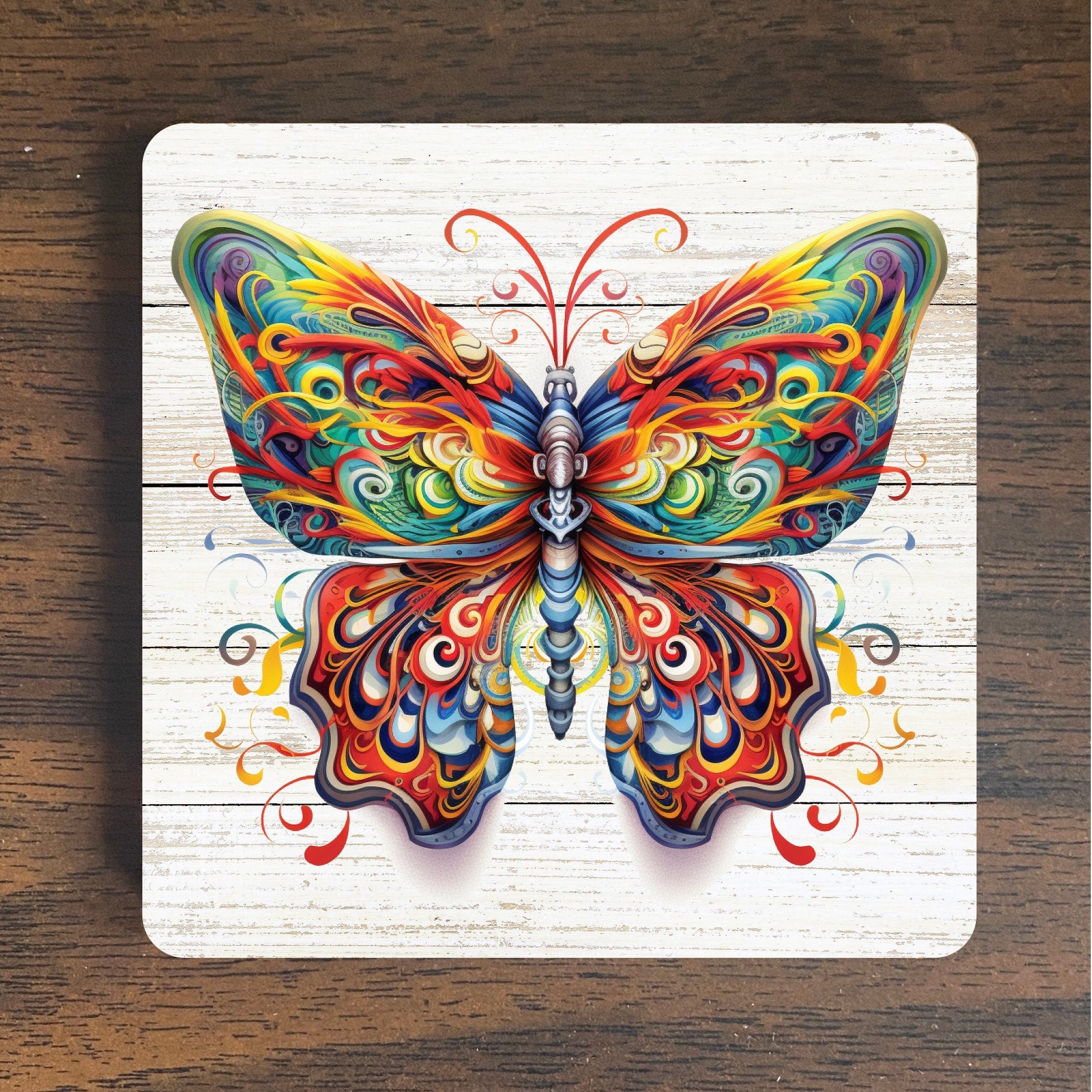The image features a vibrant, rainbow-colored butterfly artwork painted on a white wooden surface composed of five interconnected panels. The butterfly, which dominates the space, boasts intricate and swirly details, with primary colors of red, yellow, and blue, alongside shades of green, purple, pink, peach, and orange. The thorax of the butterfly is a striking blue with a metallic or armored appearance, while the antennae, six in total, are red and gracefully curling upwards from the head. This artwork, reminiscent of a tattoo, sits on a dark brown wooden table, enhancing the contrast and making the colors of the butterfly even more vivid and eye-catching.